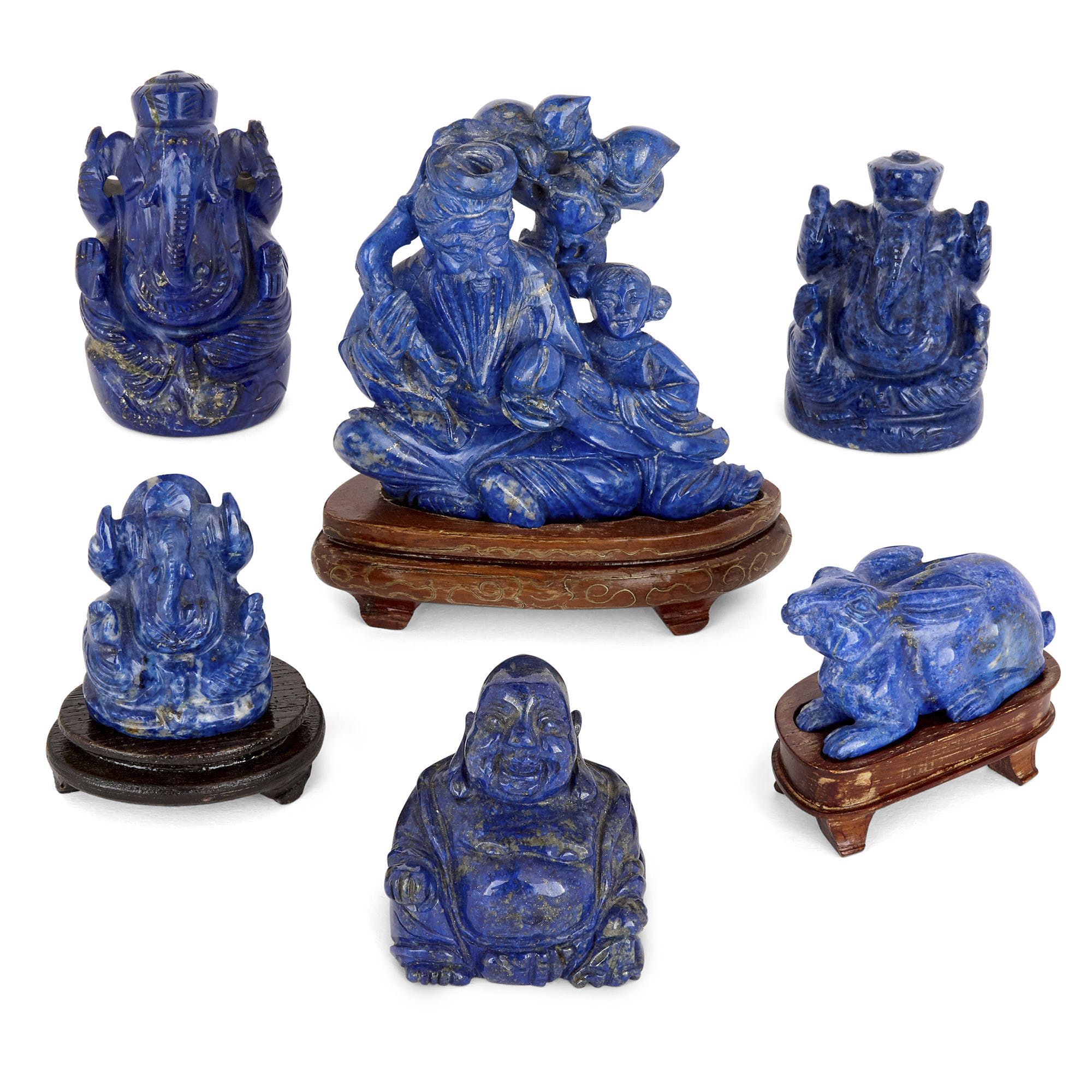A full-color photograph showcases six intricately carved blue stone statues arranged in a squarish, borderless layout against a white background. Three of the sculptures rest on wooden bases while the other three do not. The figures include: 
1. The elephant-headed god Ganesh in the upper left.
2. A bearded man, likely Confucius, seated with a small child holding his hand in the top center.
3. Another Ganesh figure in the middle left.
4. The traditional fat Buddha in the bottom center.
5. A blue rabbit in the bottom right.
6. The statue in the upper right is indistinct and its identity unclear. 

The statues appear to be crafted from lapis lazuli or possibly clay covered in blue paint, and they feature a mix of human and animal forms, reflecting themes of Buddhist and East Asian influence.